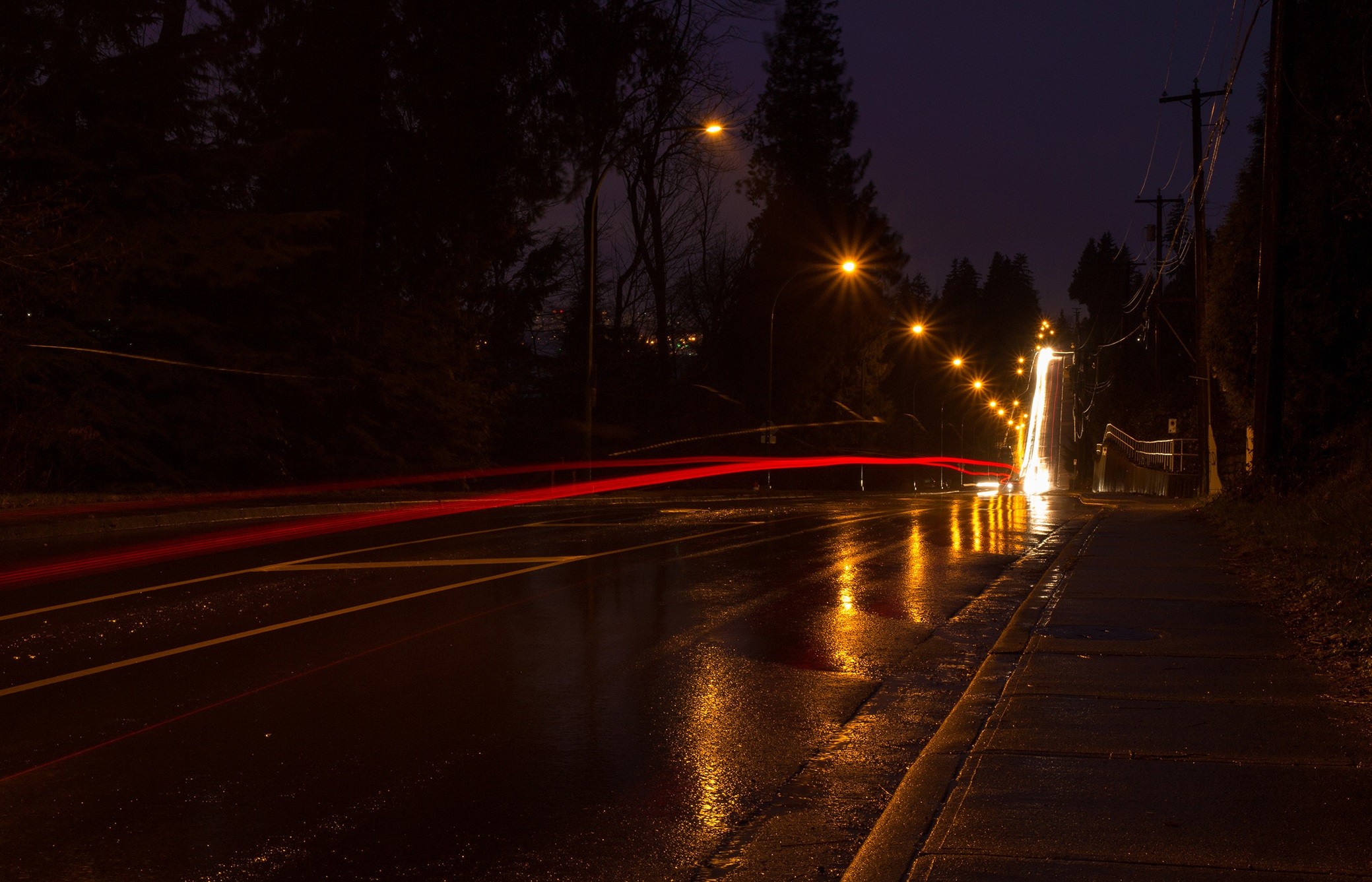This is a vivid, time-lapse photograph capturing a wet, nighttime street scene. The image shows the road starting from the left, descending a hill toward the right, and ascending another hill in the distance. The dark, rain-soaked road reflects the streaks of red brake lights and white headlights, creating a dynamic effect as if the camera's shutter speed was slowed to capture this motion. The background features a dark purple sky with a faint glow, and scattered lights from buildings peek through the silhouettes of trees. Multiple golden street lamps line the road, casting a warm light on the wet surface and enhancing the atmospheric mood of the scene. The absence of people and the blur of lights give it an ethereal, almost otherworldly quality.